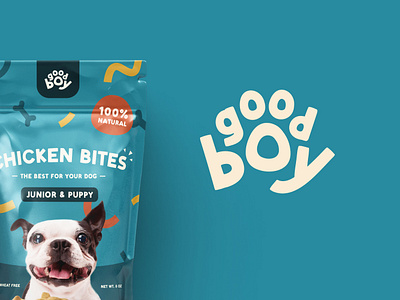This image is an advertisement for dog treats. The focal point is a teal-colored, resealable pouch prominently featuring the branding and product details. The package, which closely resembles a Ziploc bag, is set against a matching blue background. 

On the right side of the bag, the brand name "Good Boy" is displayed in large, white bubble letters, both at the top in a navy blue box and on the bag itself. 

The treats are labeled as "Chicken Bites" in large white letters positioned at the top of the pouch. Beneath this, a vibrant orange circle houses the text "100% Natural." Another prominent label in a blue box reads "Junior and Puppy," indicating the product's target demographic. Below this label, the net weight is indicated, though the exact detail is small and hard to read.

The package also features an image of a white dog with a black patch around its eyes and black ears, its mouth playfully open. The background design includes festive streamers in yellow, orange, and blue hues, adding a lively touch to the visual presentation.